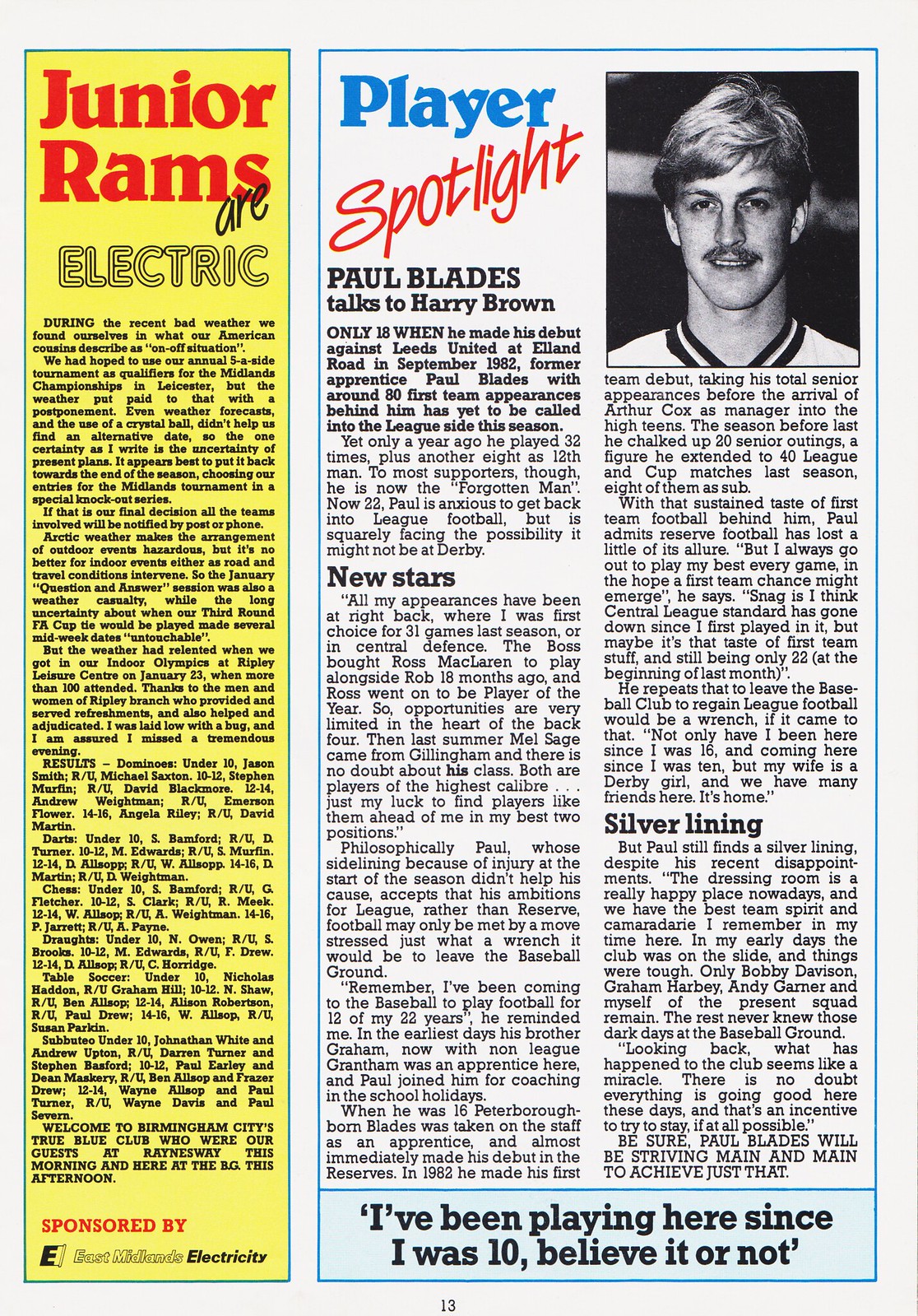The image is a scanned page from a sports-related magazine, numbered "13" at the bottom. The page is divided into three columns. The leftmost column features an article titled "Junior Rams Are Electric," displayed in black text on a yellow background. The first sentence reads, "During the recent bad weather, we found ourselves in what our American cousins describe as an on-off situation."

Adjacent to this article is a double-wide section consisting of two columns dedicated to a "Player Spotlight" on Paul Blades, with the headline reading, "Player Spotlight: Paul Blades talks to Harry Brown." The opening sentence states, "Only 18 when he made his debut against Leeds United at Elland Road in September of 1982, former apprentice Paul Blades, with around 80 first team appearances behind him, has yet to be called into the league side this season."

Beneath this headline is a detailed black-and-white portrait of a young man, presumably Paul Blades. He sports a mustache, short hair, and a jersey, and faces the camera with a smile. The text below includes additional sections labeled "new stars" and "silver lining." The left column under "Player Spotlight" is pure text, while the right column also features the photograph of Blades at the top, followed by more text.